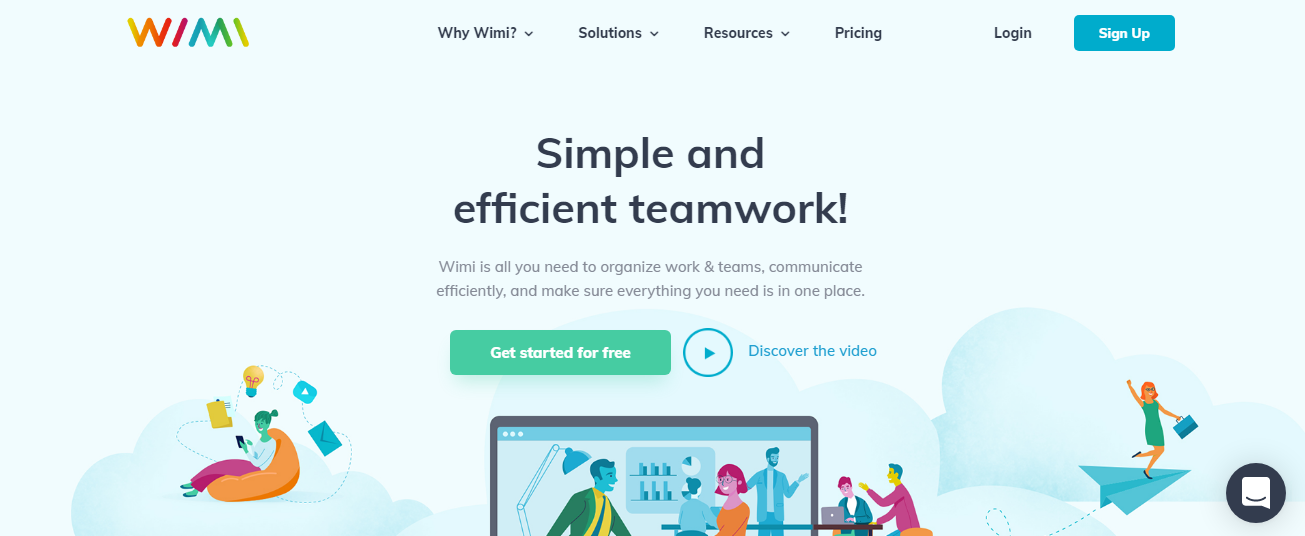Screenshot of the WIMI Webpage:

The screenshot captures the homepage of WIMI, a web-based platform designed to enhance teamwork and communication. At the top of the page is a navigation menu, featuring the following options:

- "Why WIMI?" accompanied by a down arrow for a dropdown menu
- "Solutions" with a down arrow indicating more selections
- "Resources" also with a dropdown arrow
- "Pricing" without a dropdown option
- "Login"
- "Sign Up"

The central section of the page prominently showcases a welcoming message: "Simple and efficient teamwork. WIMI is all you need to organize work in teams, communicate efficiently, and make sure everything you need is in one place." Below this message, there is a call-to-action button labeled "Get Started for Free" and an icon of an arrow within a circular button inscribed with "Discover the Video."

Scattered across the page are illustrative clip arts depicting various team collaboration scenarios. These include team members working from home, collaborating in an office environment, and engaging in teamwork while on the go.